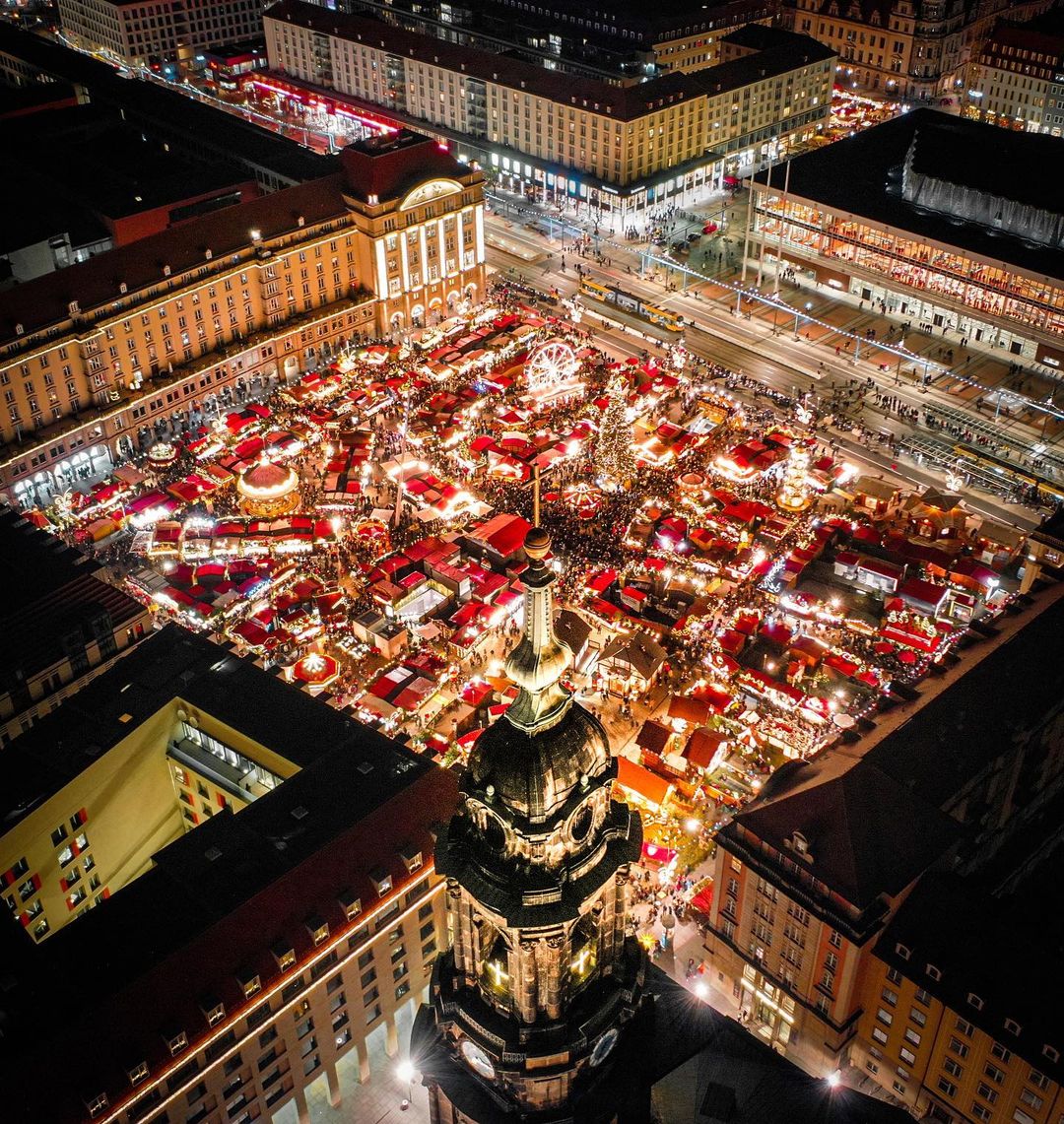The aerial photograph captures a vibrant European city square at night, illuminated for a significant celebration. The square is bustling with activity, featuring numerous vendor stalls adorned with red canopies, amusement rides including a Ferris wheel and a merry-go-round, and an array of twinkling lights. Encircling the square are tall, architecturally diverse buildings, some of which have red roofs, adding to the festive atmosphere. Dominating the foreground is a large, ornate Catholic basilica with a prominent steeple crowned by a glowing cross and smaller crosses in the cupola windows below. This dynamic scene, teeming with visitors, highlights the lively and communal spirit of the nighttime festival in the heart of this European city center.